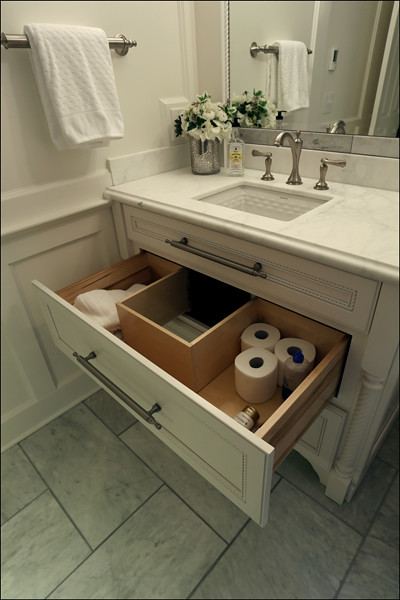The image depicts the interior of a bathroom characterized by white walls and a marble white countertop. Below the sink, there is a series of drawers featuring sleek, elongated silver-gray handles. The middle drawer is open, revealing three rolls on the right side and a piece of white fabric on the left. Atop the countertop, there is a small floral arrangement in a silver pot, showcasing white flowers. To the right and slightly in front of the floral arrangement, a clear bottle containing an unspecified liquid is visible. The overall aesthetic of the bathroom is clean and modern, accentuated by the combination of white and metallic elements.